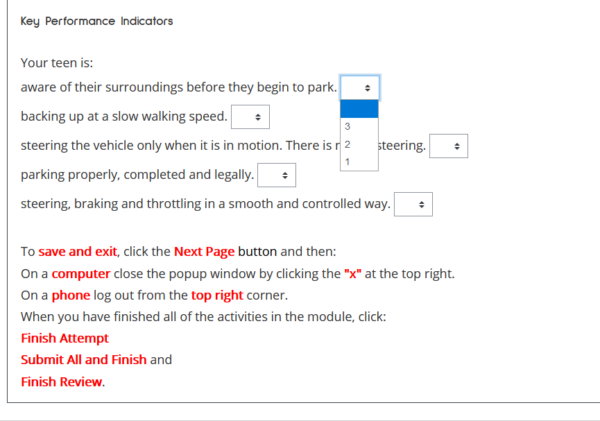In this screenshot, we observe a gray vertical line running along the left side, intersected by a horizontal gray line. Within this structured layout, the top line features bold gray text that reads, "Key Performance Indicators."

Below this heading, regular gray text outlines the following list of key performance indicators for parking, each accompanied by a pull-down box for selection:

1. "Your teen is aware of their surroundings before they begin to park."
2. "Backing up at a slow walking speed."
3. "Steering the vehicle only when it is in motion."
4. "Parking properly completed and legally."
5. "Steering, braking, and throttling in a smooth and controlled way."

Further down, there is an instructional message formatted in gray text, explaining how to save and exit the page: "To save and exit, click the 'Next' button. On a computer, close the pop-up window by clicking the 'X' at the top right. On a phone, log out from the top right corner." The overall layout presents a clean and organized visual structure that guides the user through evaluating and confirming key performance indicators.